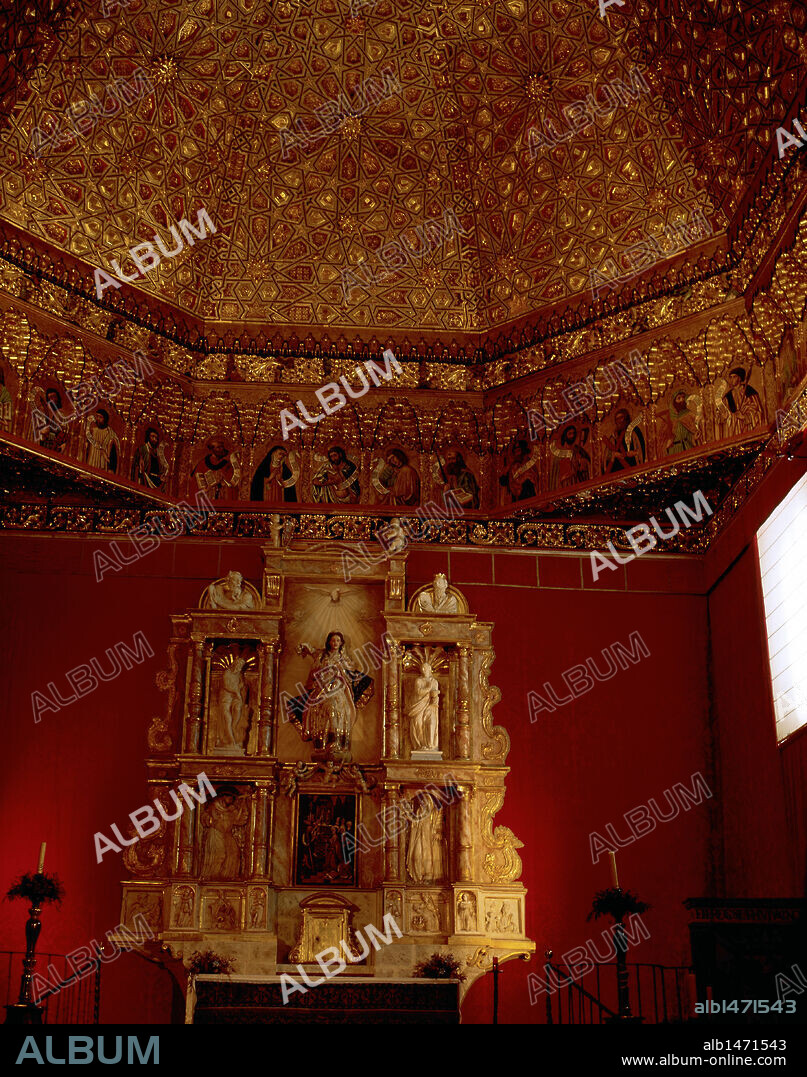The photograph depicts the interior of a richly adorned prayer shrine or temple, likely within a Catholic church. Central to the image is a gold shrine featuring three statuettes representing saints, positioned against a back wall painted in a dark reddish hue. The shrine is flanked by two prominent black candlesticks, each supporting an unlit white candle. Below the shrine, there's a small altar meant for offerings and prayer, complete with incense holders. The ceiling above showcases an intricate and ornate design, adorned with gold lacing, stars, crescent shapes, circles, and various saintly faces. Various watermarks reading "Album" and the website "www.albone-online.com" are visible across the image, indicating its origin. Additionally, the serial number ALB 1471543 is present in the bottom right corner. This elaborate scene of religious reverence highlights the skilled craftsmanship and deep spiritual significance embedded in the space.